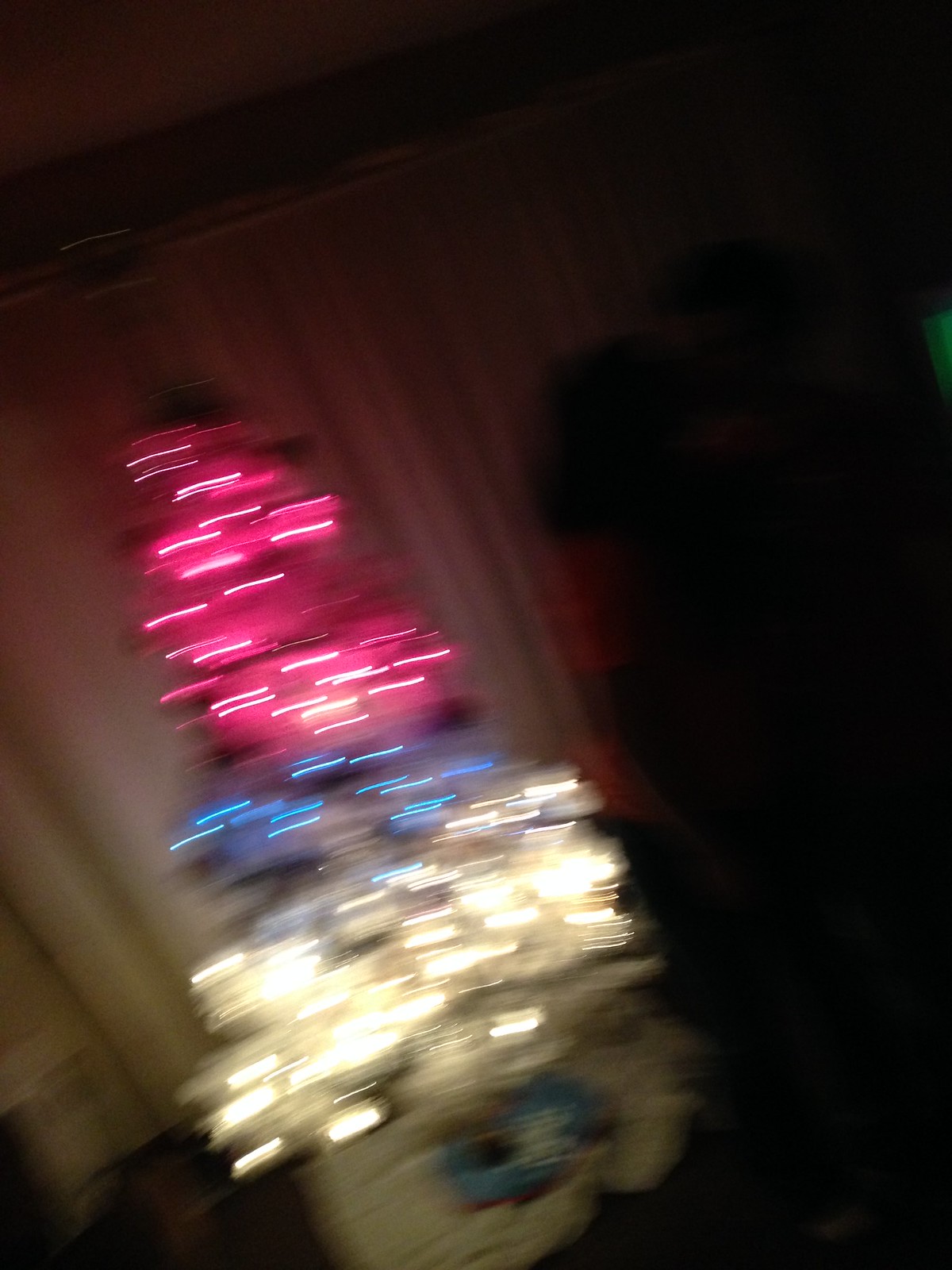In this somewhat blurry image, a small tabletop Christmas tree is prominently displayed in the background. The tree is adorned with a gradient of colorful lights; pink lights illuminate the top portion, transitioning to a middle layer of blue lights, and culminating in white lights at the bottom. Behind the festively lit tree, off-white curtains hang from a window, creating a soft backdrop. Additionally, the faint, dark shadows of two individuals standing face-to-face can be discerned in the background, giving the scene a sense of quiet intimacy. These figures appear to be dressed in dark clothing, adding to the contrast and depth of the image.